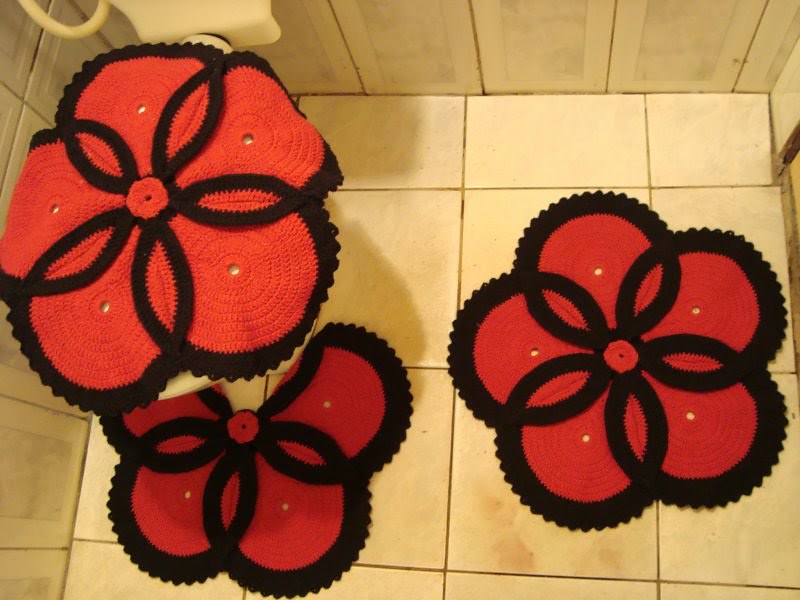The image depicts a bird's-eye view of a bathroom floor with yellowish-beige tiles, some of which show imperfections and discolored grout. The tiling is unevenly cut and extends up the wall. In the upper left corner, there’s a towel holder with a towel hanging from it. A prominent feature of the scene is the large crocheted decorations that resemble flowers. These decorations consist of five bright red circles, each bordered with black trim and featuring a red center, giving the impression of a flower with "teeth." One of these crocheted objects is draped over the toilet seat, hiding it from view. The floor has two more identical crocheted flower decorations; one is positioned around the base of the toilet, with sections cut out to fit, while another lies flat on the floor nearby. Dark spots and marks on the tiles add to the details of the scene, along with visible pipes running behind the toilet.